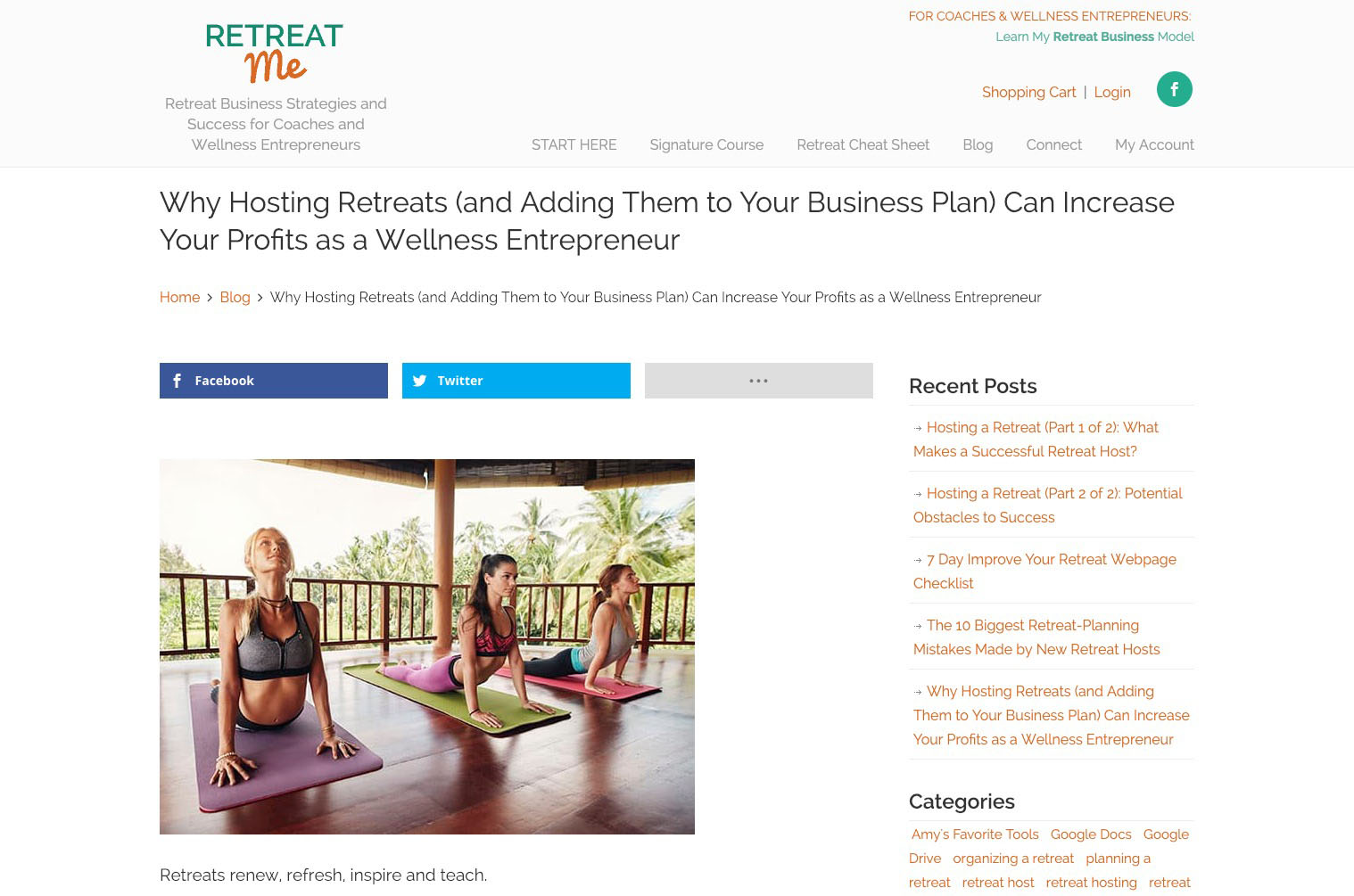**Website Screenshot Description:**

At the top left corner of the website, the logo "Retreat Me" is displayed, with "Retreat" written in green and "Me" in a shade of orangey red. Below the logo, the tagline reads: "Retreat Business Strategies and Success for Coaches and Wellness Entrepreneurs." The top navigation bar includes links for "Start Here," "Signature Course," "Retreat Cheat Sheet," "Blog," "Connect," and "My Account." On the top right corner, there are icons and links for a shopping cart, login, and a green button that appears to be for social media integration, though it is unclear if it is for Facebook or another platform.

Centrally located is a screenshot of a serene image featuring three women lying on yoga mats. They are positioned on their bellies, gazing upwards in a stretching pose. Each woman is on a different colored mat: the first on a purple mat, the second on a green mat, and the third on a pink mat. They are dressed in gym attire. The scene is set on a wooden floor, with a fenced backdrop, an open ceiling supported by poles, and trees visible in the background, suggesting an outdoor or semi-outdoor retreat setting.

The main headline on the webpage states: "Why Hosting Retreats and Adding Them to Your Business Plan Can Increase Your Profits as a Wellness Entrepreneur." Below the headline, there are more navigation links: "Home," "Blog," and quick access to social media links for Facebook and Twitter, as well as an additional menu represented by three dots.

Underneath the central image, a caption reads: "Retreats Renew, Refresh, Inspire, and Teach." To the right of the image is a list of recent blog posts. The blog entries include: 

1. "Hosting Retreat Part 2 of 2: What Makes a Successful Retreat Host."
2. "Hosting Retreat Part 2 of 2: Potential Obstacles to Success."
3. "Hosting Retreat Part 1 of 2."
4. "Seven Day Improve Your Retreat Webpage Checklist."
5. "The 10 Biggest Retreat Planning Mistakes Made by New Retreat Hosts."
6. "Why Hosting Retreats and Adding Them to Your Business Can Increase Your Profits as a Wellness Entrepreneur."

Further down the right-hand side, there is a categorized list of resources titled "Amy's Favourite Tools," which includes Google Docs, Google Drive, and various categories for planning and hosting retreats, as well as other retreat-related information. The precise details and organization of this list suggest a comprehensive resource hub for retreat-related activities and strategies.